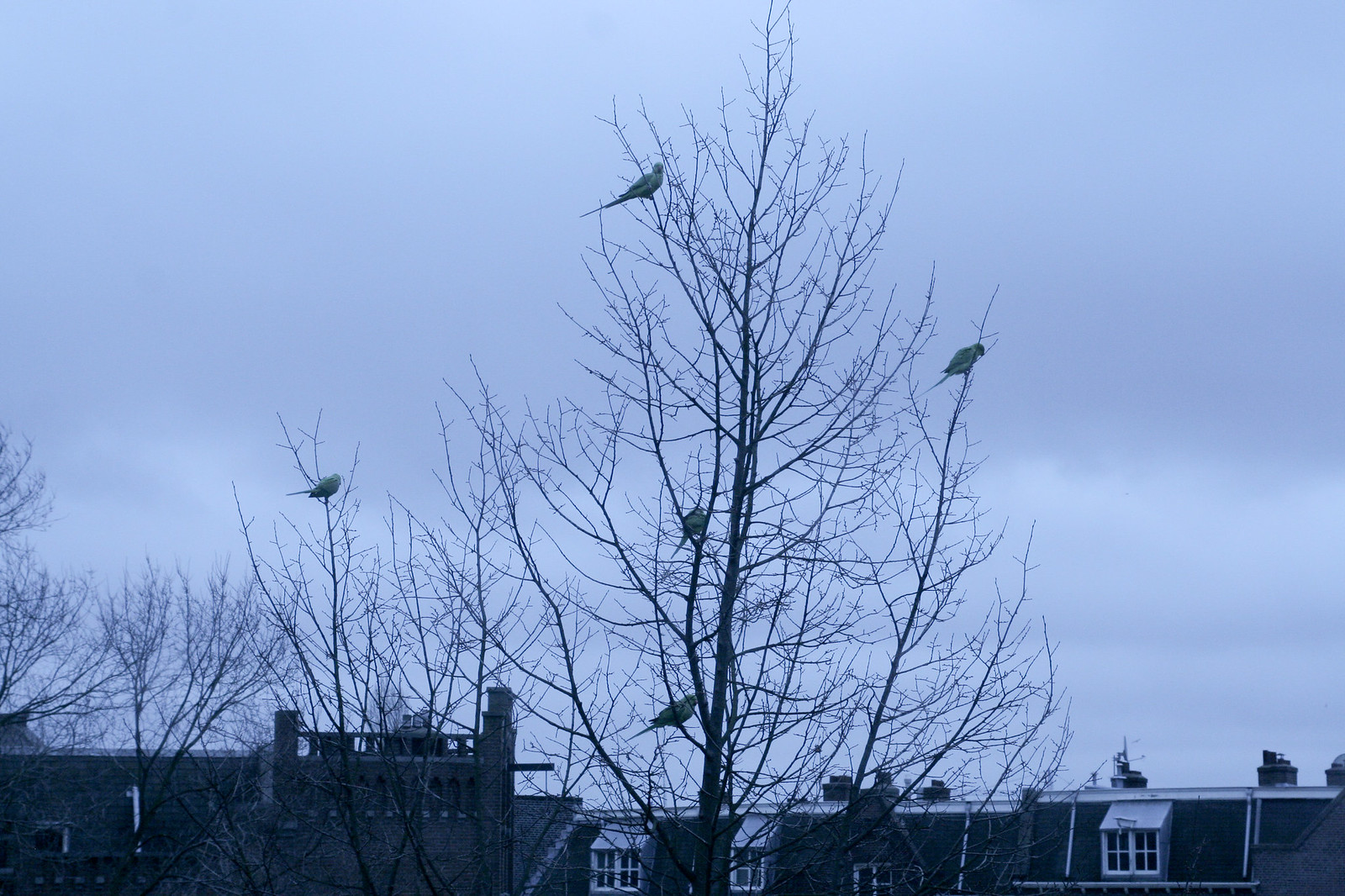The photograph features a leafless tree, likely in fall or winter, prominently positioned against a sky that transitions from blue to a dark grayish-blue, suggesting a cloudy or overcast day. The tree's bare branches serve as perches for five to six brightly colored neon green birds, which appear to be parakeets or parrots, identifiable by their curved beaks and long tail feathers. These birds display a striking color contrast, with vivid green upper feathers and white underbellies.

In the background, a cluster of buildings spans the lower part of the image. One building to the left, possibly part of an educational institution, displays ornate latticework and artistic architectural details. To the right, another building with protruding white windows is visible. The scene captures an urban setting under winter skies, with the birds providing a lively burst of color amidst the stark, leafless branches and the subdued tones of the buildings and sky.